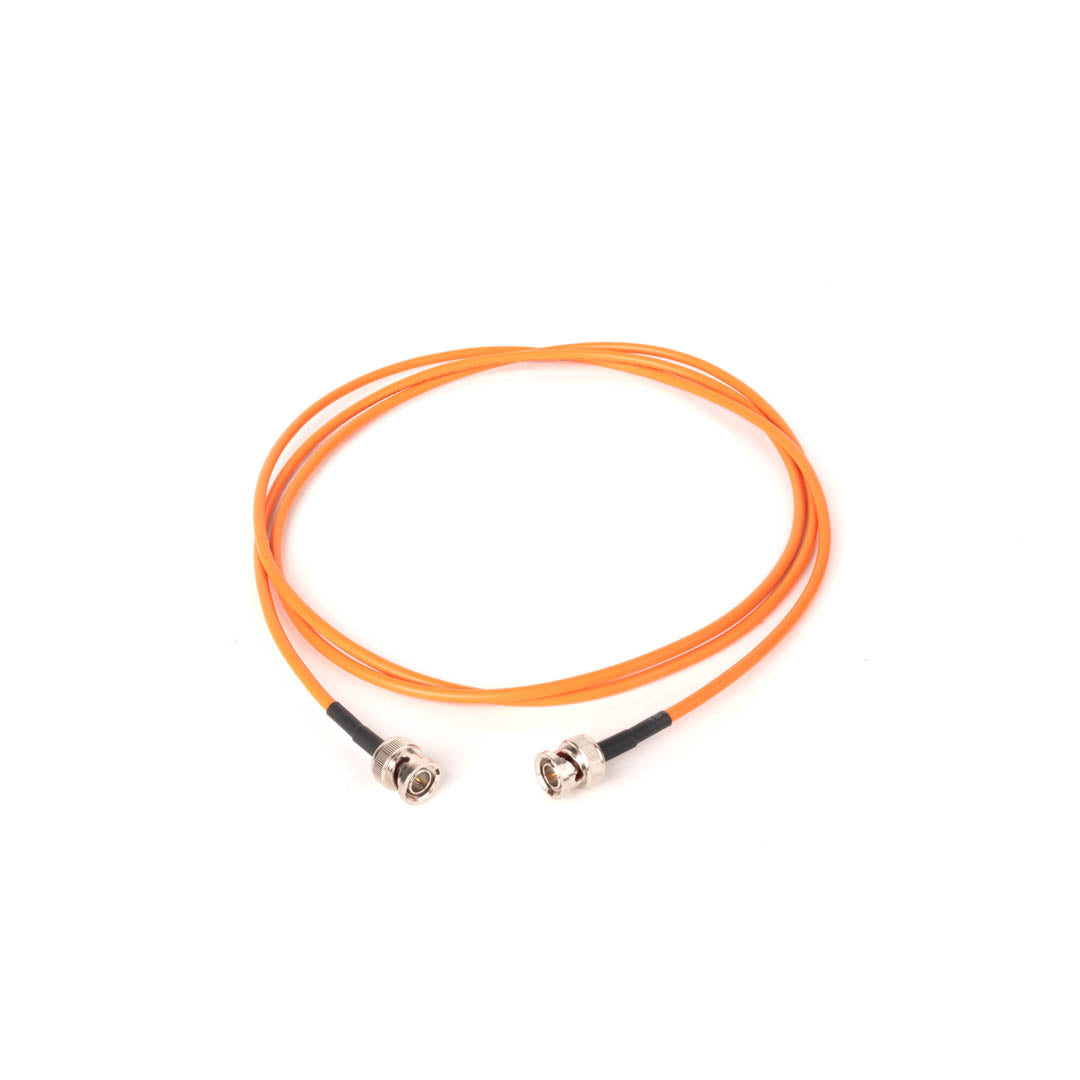This image depicts a coiled orange coaxial cable lying on a white surface. The cable, which is wound over itself three times, features black insulation near each end, transitioning into a brushed nickel or chrome cylindrical fitting. Each end of the cable boasts a distinct fitting design: one end has a bolt for screwing, while the other is smooth and round, suggesting a push-in or screw-in mechanism. Both ends are male connectors with visible pins inside the fittings. The fittings are narrower at the tips and feature black borders at the base, where they meet the orange coating of the cable. The entire setup is neatly arranged in a circular formation in the middle of the table.